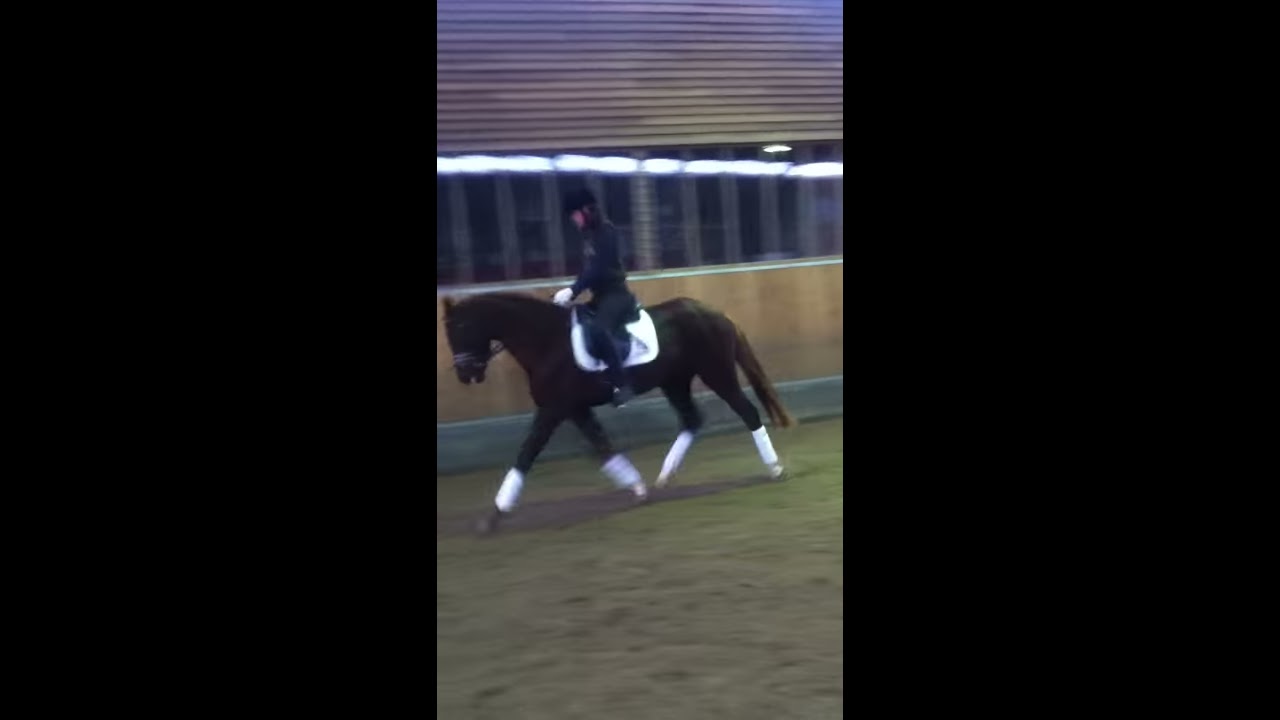In this detailed image, a female jockey is riding a dark brown horse with distinctive white markings on its lower legs, possibly protective wraps or socks. She is clad in a traditional equestrian outfit, predominantly black, including black pants, a long-sleeve shirt, appropriate riding footwear, and a black helmet that secures her brown hair. Notably, she wears white gloves that stand out against her dark attire. The horse is equipped with a white saddle, and a bridle adorns its head. They are moving across a grass-covered field that has patches of dirt, suggesting an arena or outdoor training facility. In the background, there is a structure with a brown wooden roof and walls painted yellow, along with a fence on either side, indicating the presence of a controlled area for equestrian activities. The scene captures the dynamic essence of equestrian sport within a well-maintained, structured environment.